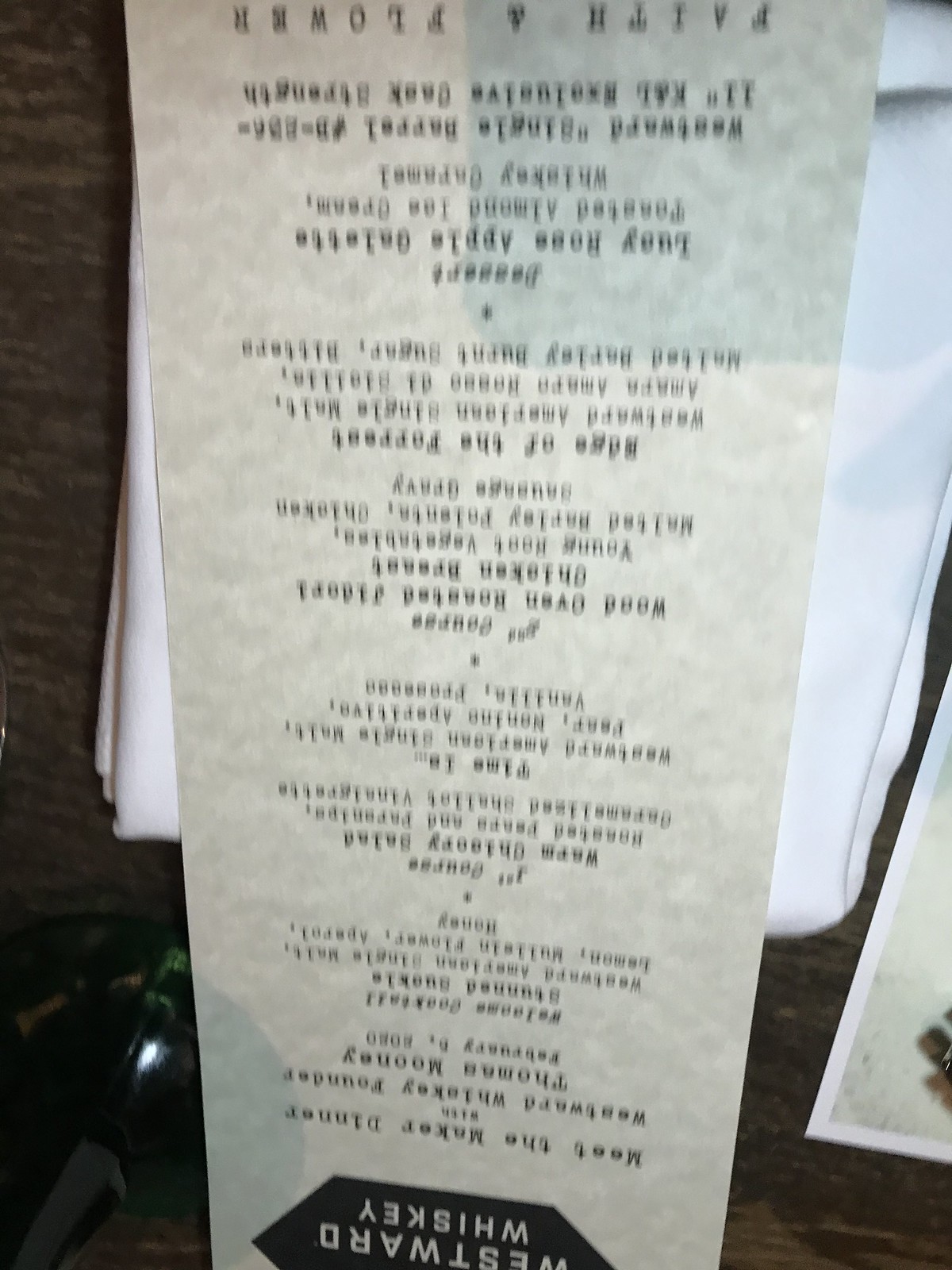An upside-down photograph captures a drinks menu with a predominantly black background and white text. At the apparent bottom of the picture, which is actually the top due to the image being upside-down, the text reads "West White Whiskey." The menu details a special event, noted as "Meet the Maker Dinner with West White Whiskey Founder, Thomas Mooney," scheduled for February 6th. Unfortunately, the year is not visible.

Further down, the section titles appear somewhat readable despite the blurriness. One paragraph lists a "Warm O'Lorry Salad, Roasted Farrah, and Farrah Pills," while another mentions "Westward American Single Wall, Fear Montagne." Another section, believed to be for dessert, is titled "Lucy Rose Apple Palette," followed by "West White Single Farrell B11 Cup." The remainder of the text is indistinct, rendering it difficult to interpret fully. The menu appears to offer a unique culinary experience themed around West White Whiskey.